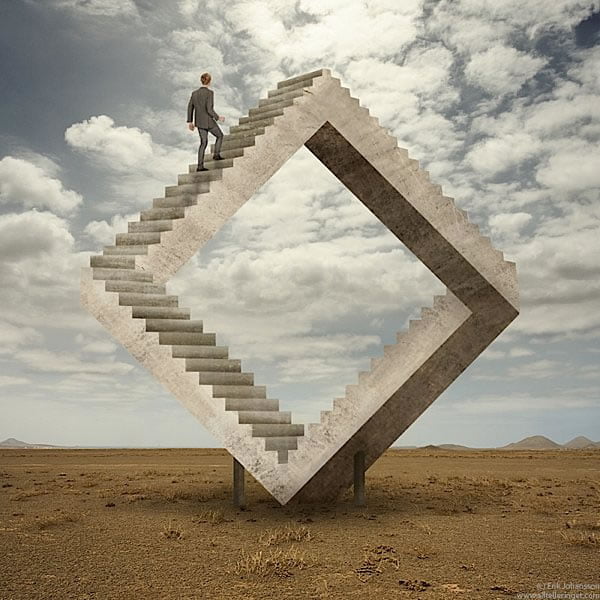The image depicts an optical illusion featuring an intricately twisted staircase made of stone or concrete, set in a barren landscape with brown dirt and distant hills or small mountains. This stairway forms a diamond shape with sections that defy the laws of physics, creating an impossible and continuous loop. The structure appears to rise diagonally to the left, then turn right and ascend further, only to descend downward and to the right in a zigzag pattern, before making another sharp turn down and left, giving the illusion that it connects endlessly. A man in a business suit is seen climbing the stairs, seemingly navigating this perplexing path. Overhead, a cloudy sky adds depth to the otherwise stark background. The artwork is skillfully detailed, with the illusion that makes the staircase appear both surreal and fascinatingly complex.